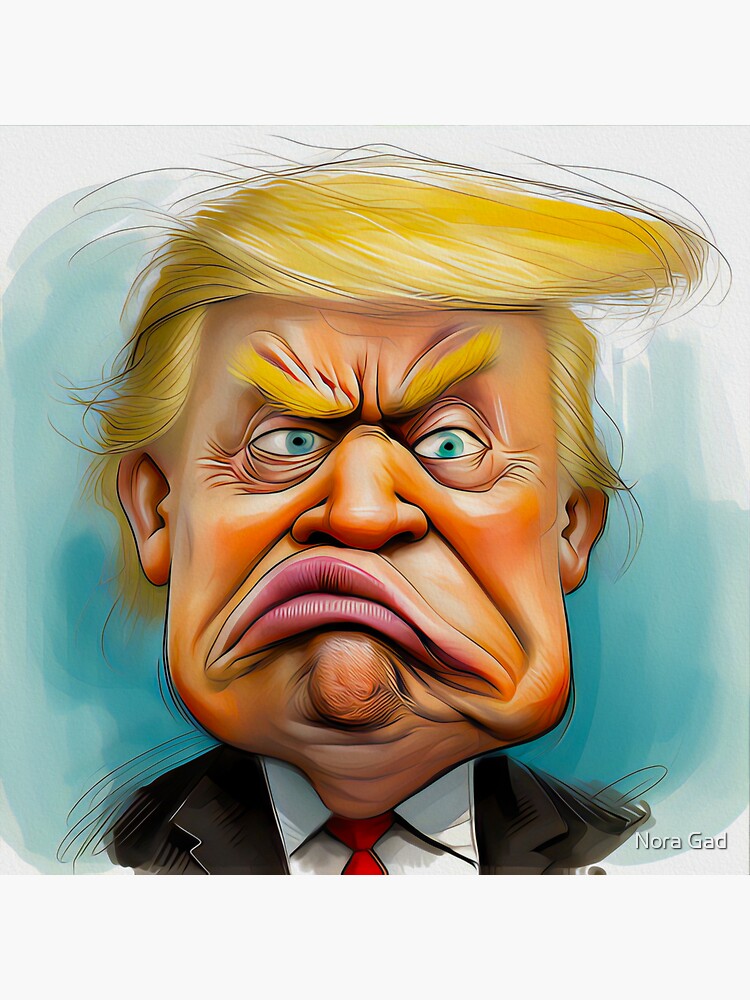This digital caricature by Nora Gadd portrays an extremely exaggerated and highly detailed image of a very angry Donald Trump. His long, prominent blonde hair, with strands distinctly separated and blowing to the left, matches his dramatically slanted blonde eyebrows. His face is characterized by deep wrinkles and crow's feet around his intensely squinting blue eyes, conveying a look of disgust. His unusually large nose and big, pouty lips form an upside-down U, emphasizing his frown. Below his bulbous chin and heavily jowled neck, he wears a formal suit marked by a red tie, white collared shirt, and black jacket. The background features two shades of blue, transitioning seamlessly to white, adding depth to the composition. The image is signed at the bottom right with the artist's printed name, Nora Gadd.